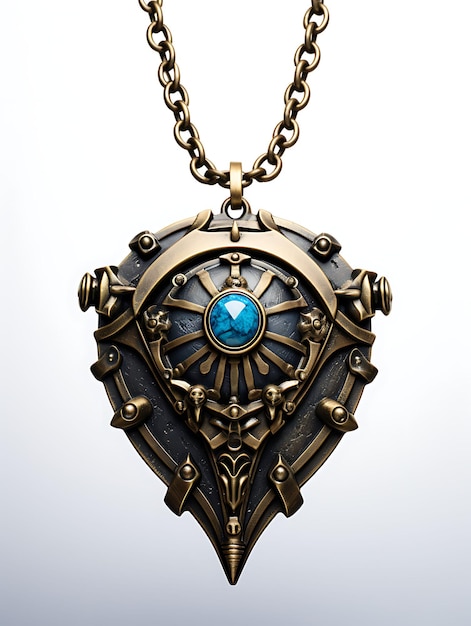This image showcases a pendant hanging from a heavy, brass-colored chain with sizable links. The pendant, teardrop-shaped and adorned with intricate metal markings, has a blue stone at its center. Lines radiate outward from the stone, forming a circular pattern that encircles two small skulls positioned beneath the stone. The pendant narrows down to a point, creating a harmonious but striking contrast between the blue gemstone and the bronze hued accents, with subtle hints of black enhancing the overall antiquated appearance of the jewelry piece.